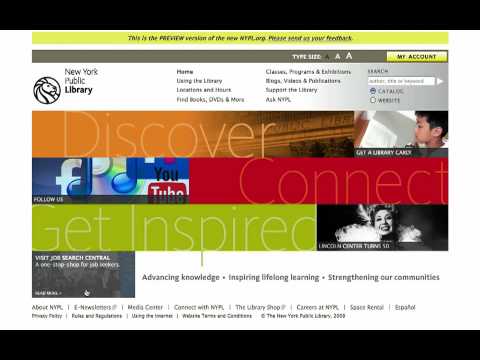The webpage features a vibrant and dynamic layout with multiple color-themed sections, both at the top and bottom, with striking black banners. 

At the top, a lime green banner leaning towards yellow is present, although the text within it is slightly blurred and difficult to decipher. Beneath this, a white space transitions into a mushroom-colored banner, which houses text related to font size. This section includes three icons: a small black "A," a medium white "A," and a large white "A."

Proceeding downward, there is a fluorescent yellow banner with black text that reads "My Account." Following this, a tan banner prominently displays "New York Public Library." This section contains navigational links: "Home," "About the Library," "Support the Library," "Classes," "Ask," and a search bar.

Further down, an orange banner boldly announces "Discover," succeeded by a red banner with the word "Connect." Finally, a green banner encourages users to "Get Inspired." Below these banners, phrases like "Advanced Knowledge," "Inspiring Lifelong Learning," and "Strengthening Our Communities" emphasize the library's mission and goals.